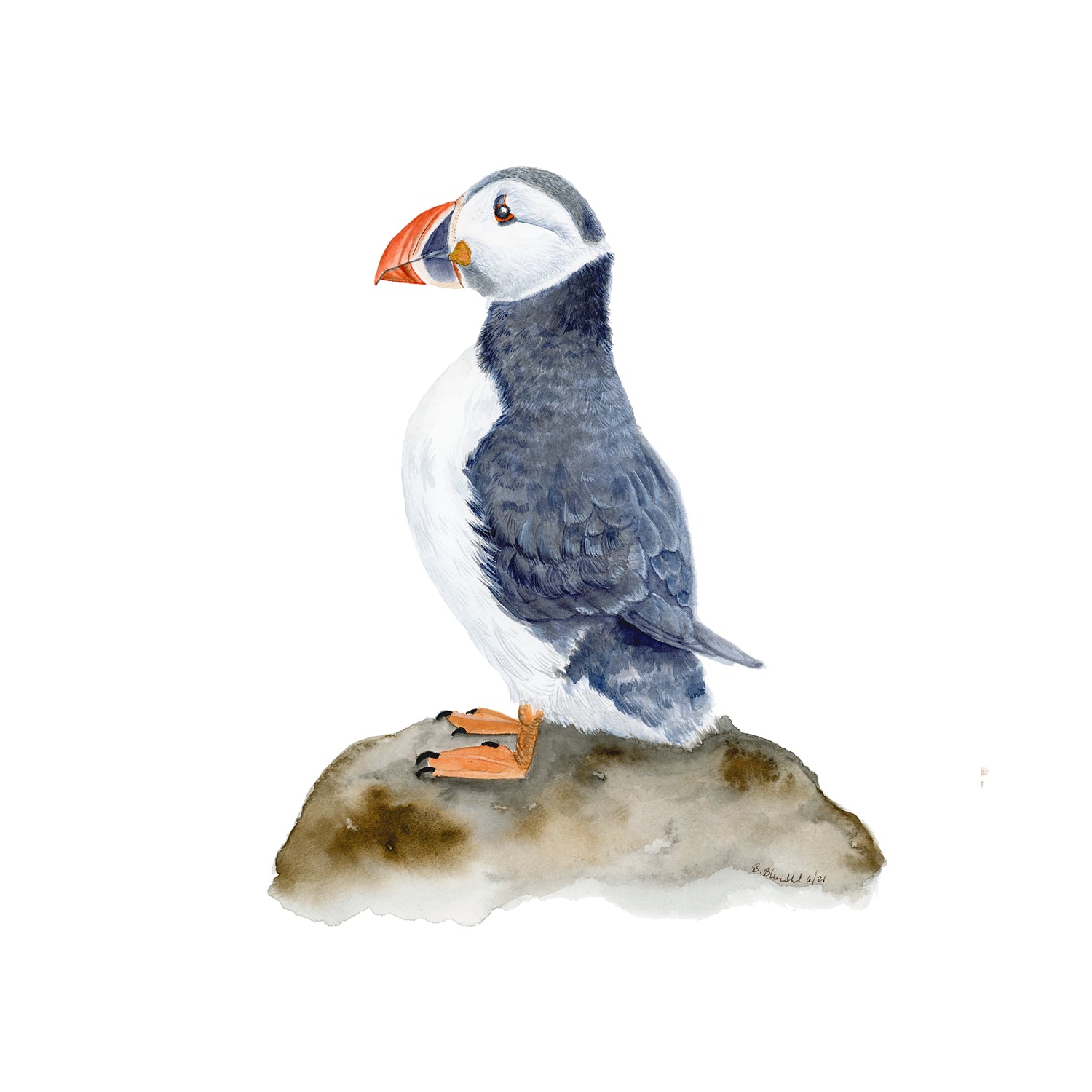The image is a detailed digital painting of a puffin standing upright on a brownish tan rock, looking slightly to the left. The puffin boasts a multicolored beak, predominantly reddish brown with white and blue accents, and dark brown eyes that appear a bit sad. Its underbelly and chest are pristine white, while its back features a complex blend of dark grayish blue and black hues. The puffin's wing, partly visible, aligns with the dark coloration of its back. Its short, stubby wings, webbed feet with three black nails each, and orange-to-brown legs further distinguish it. The bird's head is accented by a subtle black stripe, adding to its distinctive appearance. The image lacks visible text, focusing solely on the puffin and its detailed, contrasting coloration.